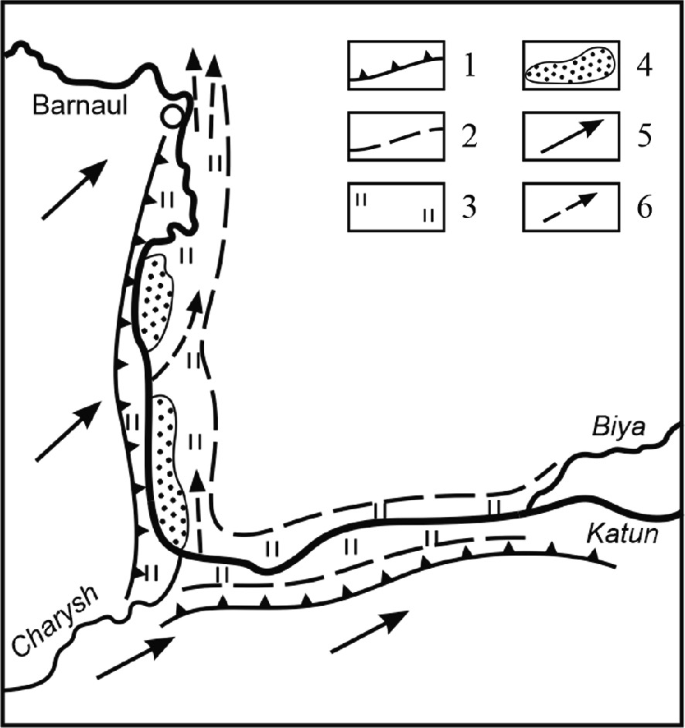The image appears to be a rudimentary, pencil-like drawing of a geographical map featuring multiple waterways. The map includes notable locations labeled "BARNAUL" at the top left, "CHARYSH" at the bottom left, "BIYA" at the bottom right, and "KATUN" right below "BiYA." Arrows throughout the map indicate directions, with a central line running from the right to the left, then upwards, and continuing left again. Surrounding this primary line are additional arrows and lines; notably, four arrows point upwards, with two additional arrows situated towards the bottom also pointing up. On the right side, two vertical lines extend from top to bottom. 

In the top right corner, there is a legend or key numbered 1 through 6, each contained within black-outlined boxes. Number one features a line with spikes, while number two is depicted as a dashed line. Number three includes two parallel lines in both the upper left and bottom right of the box. Number four showcases an irregular shape filled with black dots. Number five and six are labeled with arrows; number five is a solid arrow pointing right, and number six is a dashed arrow pointing right with a line in the middle of the stem. The background of the map is predominantly white, providing a stark contrast to the detailed black-lined drawings and annotations. The map appears to serve an educational or instructive purpose, perhaps related to geographical studies of the named regions and their watercourses.